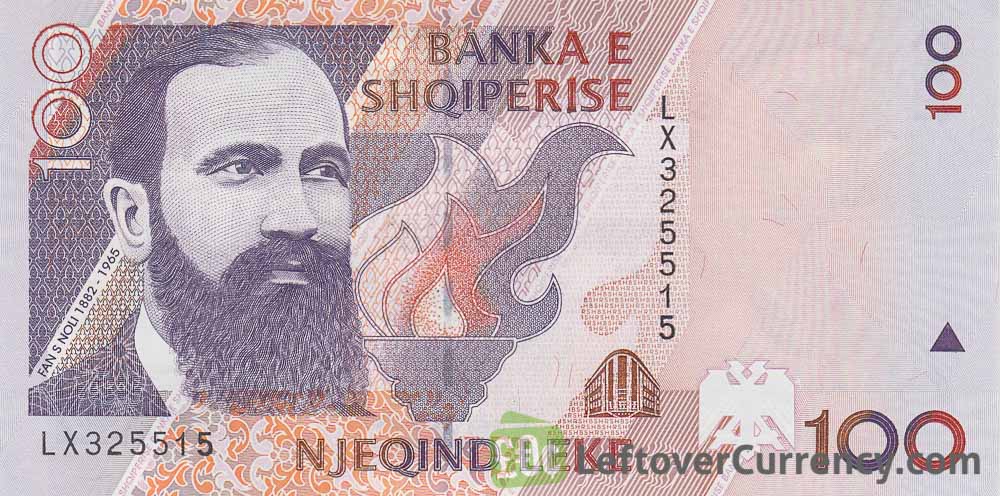This image portrays a detailed digital screenshot of foreign currency, specifically a 100-unit bill. The banknote prominently displays the text "Banka e Shqipërisë" towards the top center, indicating its origin. The number 100, signifying its value, is visible in the top left, top right, and bottom right corners. Additionally, the bottom right corner features the website "LeftoverCurrency.com."

The bill is adorned with vibrant colors, primarily orange and black, with accents of green, purple, and blue. An illustration of a distinguished man with a long beard and slicked back hair is positioned on the left side. This figure is identified as Fan S. Noli (1882-1965), whose name and lifespan are labeled beside his image. To the right of Noli, there are illustrations of a torch and an old building, further enhancing the currency's intricate design. 

This detailed depiction of the 100-unit banknote from Albania elegantly showcases its historical and artistic elements.